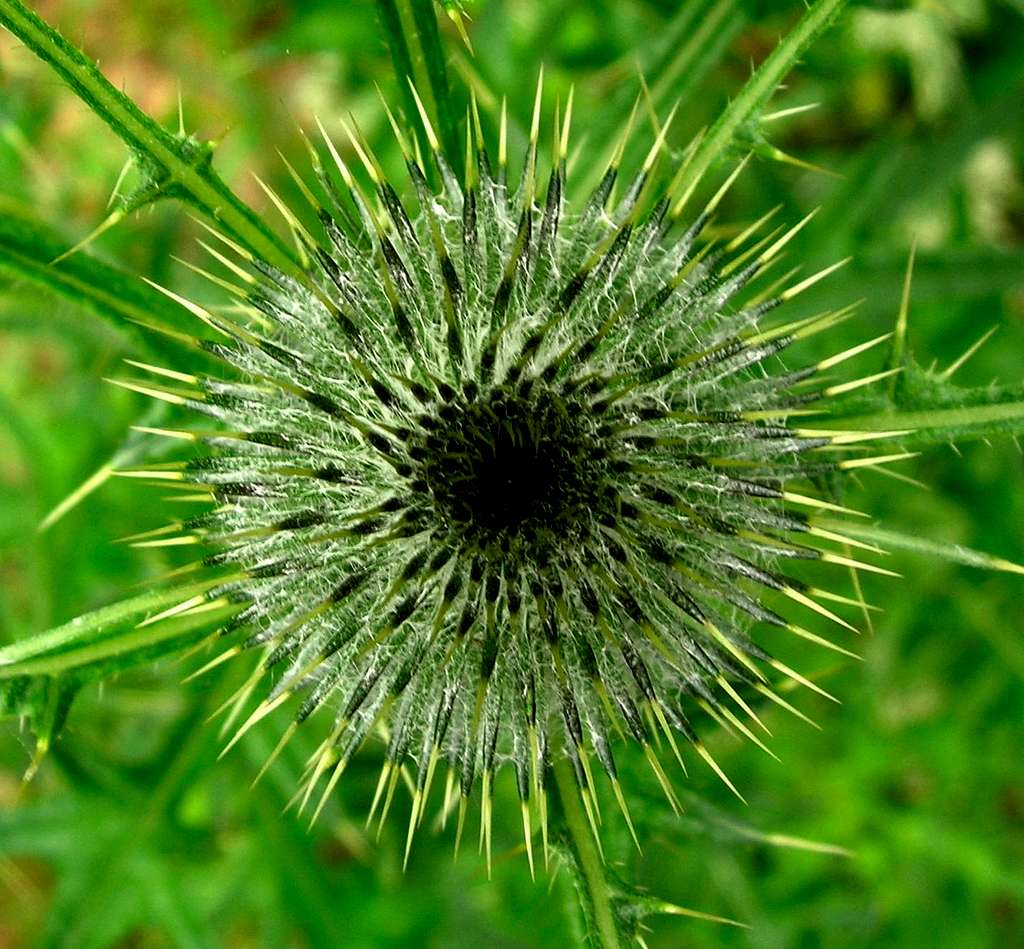This image offers a top-down, close-up view of a thistle, filling almost the entire frame and showcasing its intricate details. The photograph captures the dense black center surrounded by a mix of black, white, and gray fluffy inner petals. Spiky, light green petals extend outward, adding to the thistle's overall spiky appearance. The image focuses sharply on the top part of the thistle, revealing its unique textures, while the background remains a blurred expanse of green, hinting at additional foliage and pointy leaves. The thistle is centered in the photograph and occupies about 80% of the picture, emphasizing its striking structure against a fuzzy green backdrop.